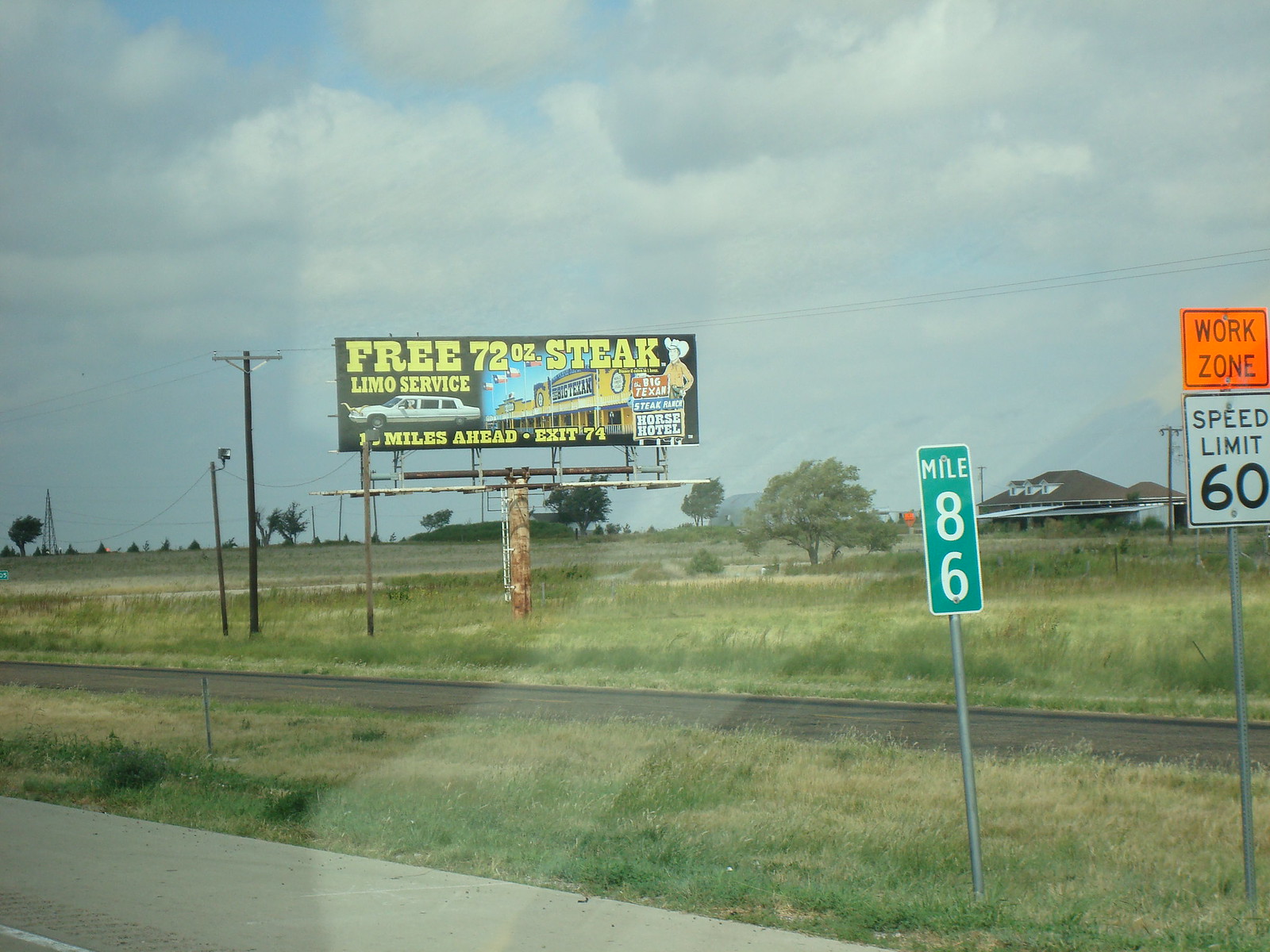This image captures a detailed and expansive roadside view taken from inside a car window, showcasing a large billboard along a Texas road, likely in the Panhandle near Amarillo. The grassy median separates the main road from a single-lane service road or unmarked blacktop. Prominently, the green mile marker sign displays "Mile 86" alongside a yellow work zone sign, beneath which is a white speed limit sign indicating 60 miles per hour.

Central to the photograph is a rusted yet vivid billboard promoting the Big Texan Steakhouse, renowned for its offer of a free 72-ounce steak and limo service. The billboard includes an illustration of a cowboy and a photograph of a yellow saloon-like building with at least four or five Texas flags on poles in front. Part of the billboard's text is obscured by a post, but it conveys that the destination is approximately 10 or 12 miles ahead near exit 74. The background includes a sprawling flat field dotted with power lines, and a ranch house can be seen off to the side, giving the scene an authentic prairie ambiance. The sky overhead appears to be very cloudy, contributing to the expansive and somewhat rustic atmosphere of this typical Texan roadside scene.